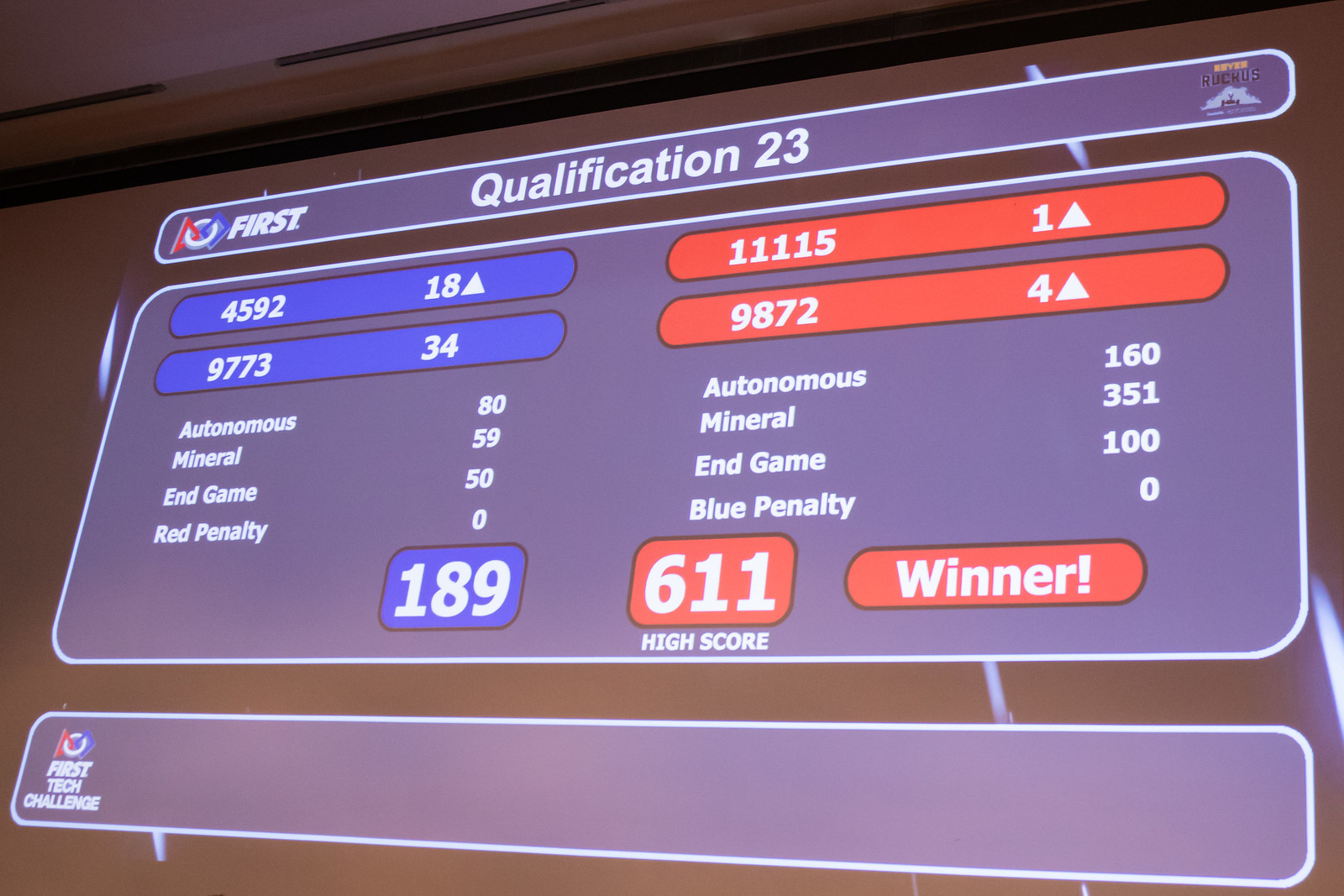The photograph captures a large billboard or projection screen, likely at a racetrack or a sporting event. Dominating the image, the screen is devoid of any people, emphasizing the display itself. At the top, it prominently reads "First Qualification 23" with a visible logo in the upper left corner indicating "First Tech Challenge," hinting at a technology-related competition, possibly a robotics challenge. Below, the text details the scores and categories: "Autonomous," "Mineral," "Endgame," along with "Red Penalty" and "Blue Penalty." The scores are distinctly displayed: Red Team with 611 points and Blue Team with 189 points, declaring the Red Team as the winner. The color scheme of the screen includes Brown, Tan, Black, White, Blue, Red, Purple, and Orange, creating a vivid and informative display.